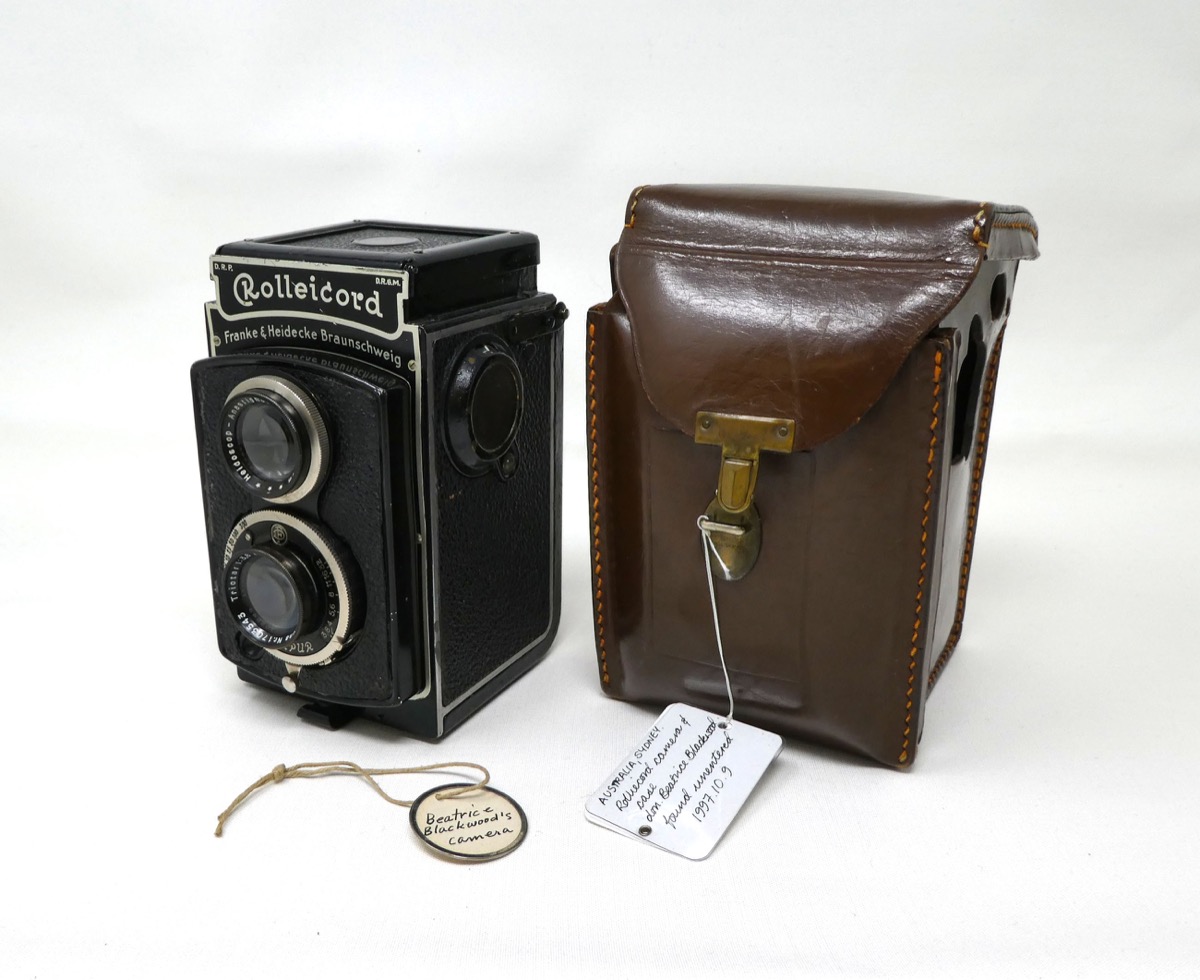In this image, set against a white background, there is an antique, boxy, black camera on the left side, which prominently features the text "Rollycord" and "Frank and Heinrich Braunschweig." The front of the camera has two lenses and a knob on the right side. Below the camera is a round, hanging tag that reads "Beatrice Blackwood's Camera." To the right of this camera is a dark brown leather case, meticulously detailed with lighter brown stitching and fastened with a brass buckle. This camera bag has a white tag tied to its fastener by a string, inscribed with "Australia, Sydney" and further illegible cursive text alongside a date: 1997-10-9. This entire composition resembles an advertisement, showcasing the vintage camera and its matching case.